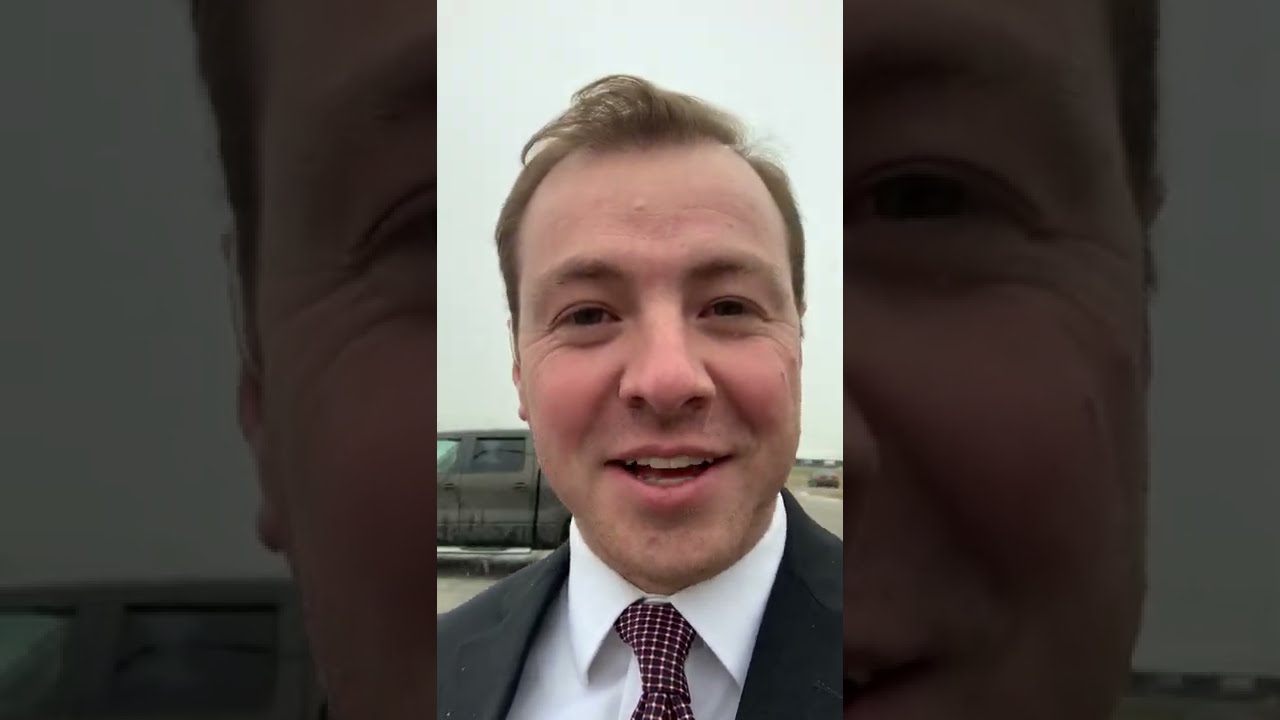The image depicts a man with auburn-brown hair that is short on the sides and swooshed to the left, standing in the center and facing the camera. He is dressed in a formal dark gray or blue suit jacket, a white collared button-down shirt, and a maroon tie with white stripes or checkered patterns. The man appears to be smiling or talking, enhancing the expression on his face. The background shows a cloudy, gray sky and a truck, which appears dirty and possibly black or green, located behind his right shoulder. The picture has good lighting and seems to be a vertical selfie taken with a cell phone, focusing closely on the man’s face while the truck remains slightly blurred. This image could also be perceived as a screenshot from a formal speech, given the man’s attire and facial expression.